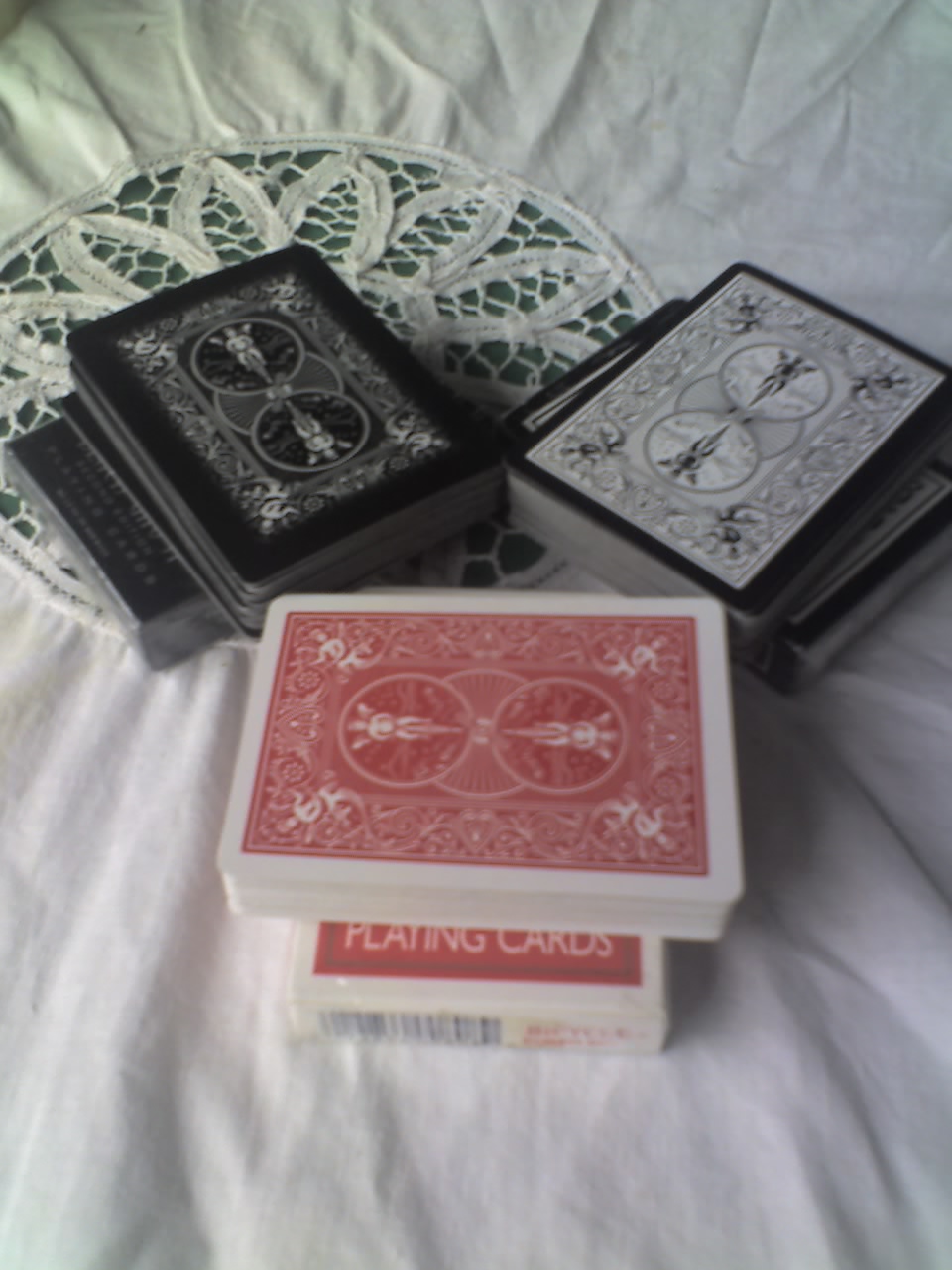The image showcases three meticulously arranged stacks of playing cards positioned on a pristine white cloth backdrop. The stack on the left features a predominantly black design adorned with intricate white, tech-inspired patterns and decorative elements. Adjacent to it, the stack on the right is mainly white but embellished with striking black geometric shapes and designs. In the foreground, beneath these two piles, is a considerably tall stack of red playing cards, creating an eye-catching contrast against the background. The overall composition highlights the diversity and intricate detailing of the playing card designs.